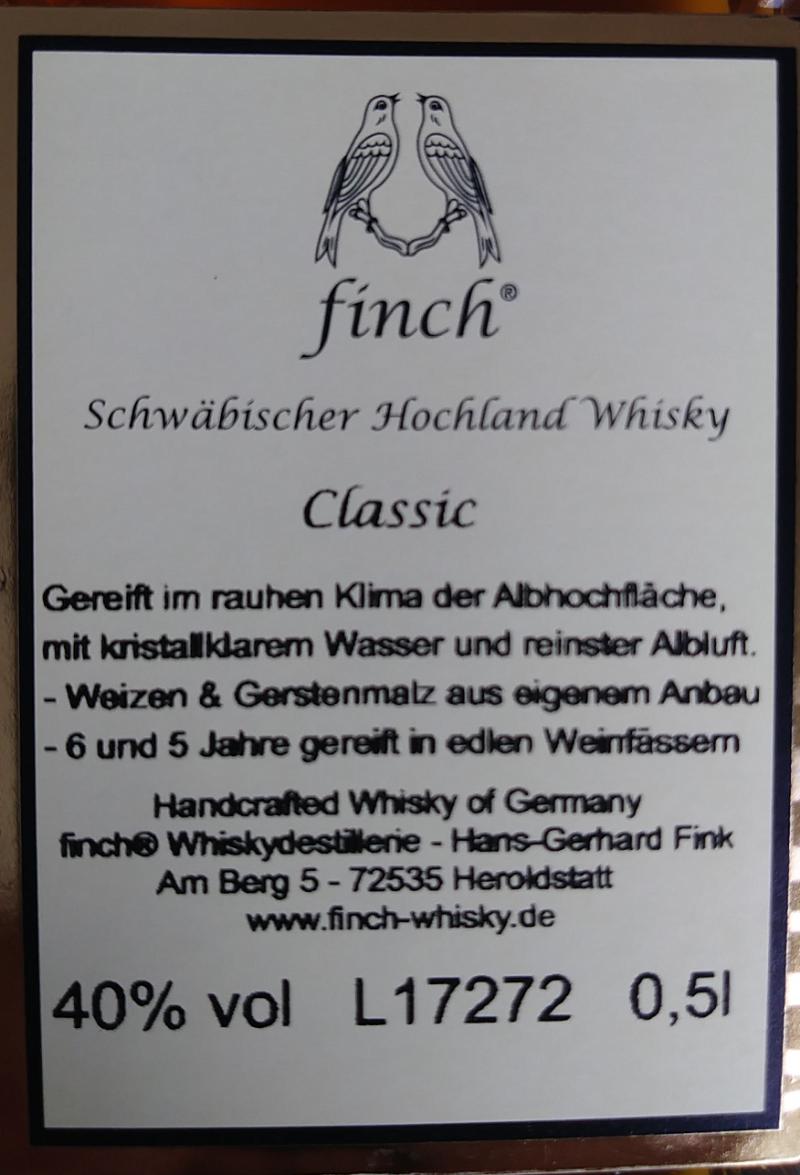The image captures an up-close view of a leaflet or label with a detailed design for Finch®, a brand of handcrafted German whiskey. The backdrop is brown, with a central white section framed by a black outline. Dominating the top portion of this label is the Finch logo, featuring two intricately drawn birds facing each other, seemingly connected through their feathers. Below the logo, in black ink, the text reads "Schwabischer Hochland Whiskey" followed by "Classic." The label includes a four-line paragraph in German, beginning with "Gereift" and ending with "Weinfassam." Further down, in bold text, it states "Handcrafted Whiskey of Germany." The label also mentions key details such as a 40% alcohol volume, the batch number L17272, a volume of 0.5 liters, and the official website, www.finch-whiskey.de. The craftsmanship of the whiskey is credited to Whiskey Destillerie Hans Gerhard Fink. This professionally designed label, free from color yet rich in detail, signifies a high-quality product.